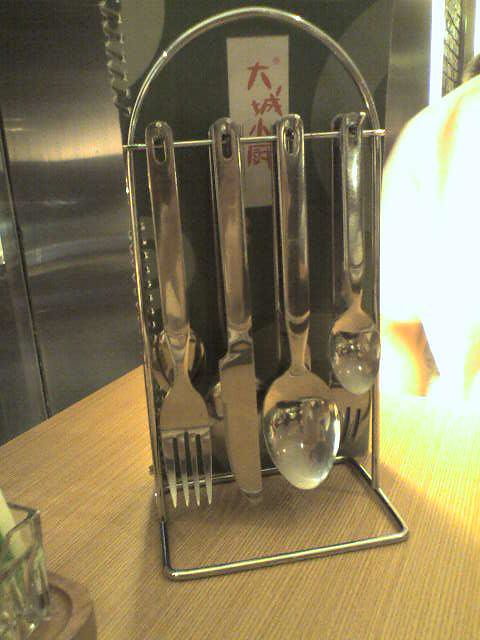The photograph showcases a detailed utensil display on a light brown wooden tabletop. The metal wire holder, fashioned from stainless steel with a square base and rounded arch top, features a central bar with hooks from which silver utensils hang. On each side, the arrangement consists of a fork, a butter knife, a tablespoon, and a teaspoon, mirrored on the reverse. Behind the holder, a white rectangle adorned with red Chinese or Japanese characters is visible, possibly part of a menu or a label. The backdrop includes a commercial stainless steel refrigerator, adding to the kitchen setting. Additional elements in the scene include a small glass container with a lime, positioned at the bottom left, and a brightly reflected light source to the right. The overall composition presents a meticulously organized kitchen space.